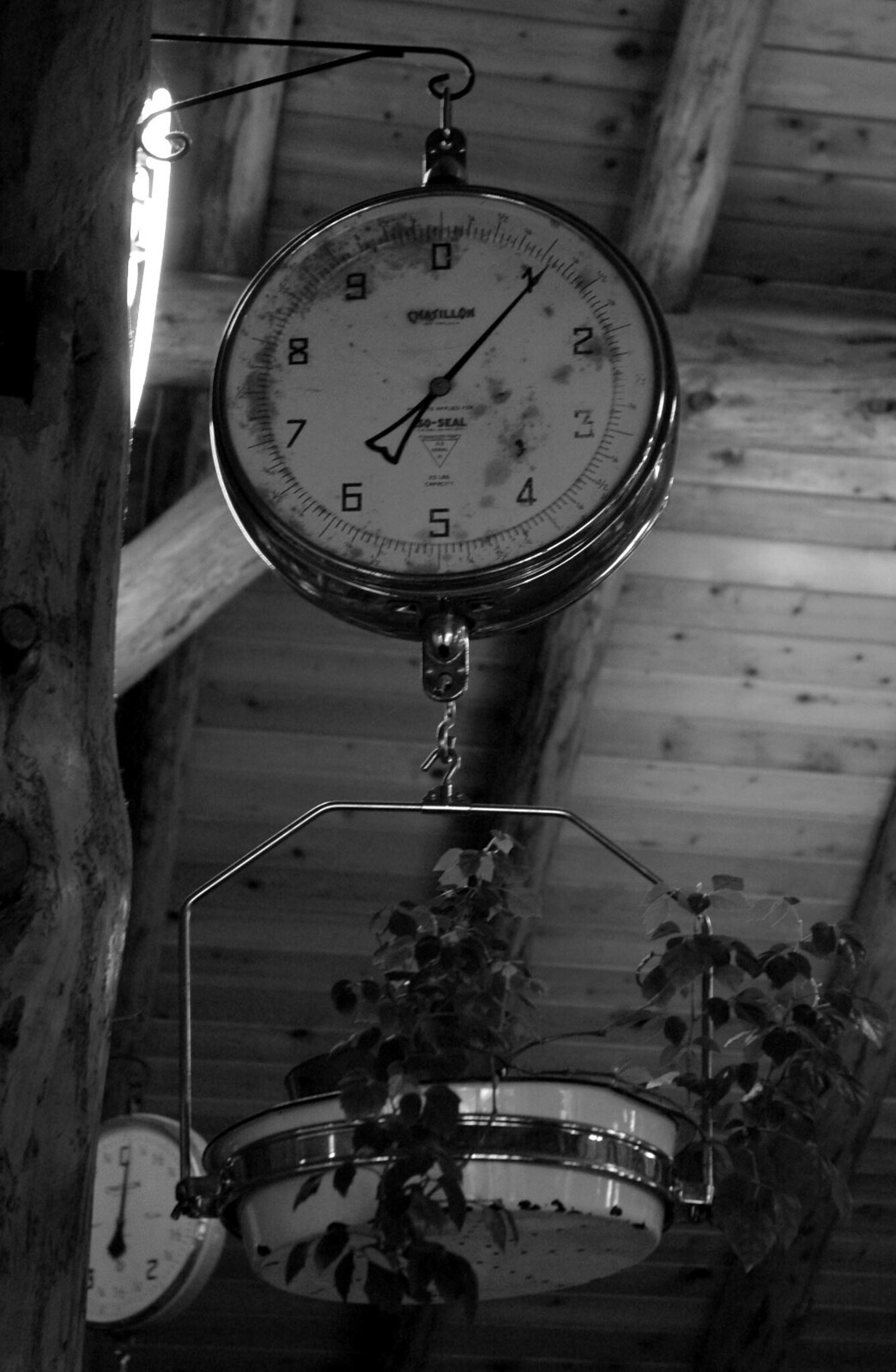This black and white photograph captures an old, likely antique, weighing scale mounted on the wall of what appears to be a rustic cabin. The image focuses on the scale, which is fixed to the wall by a black iron hook extending outwards. The scale itself is a circular device, resembling a clock, with numbers ranging from zero to ten pounds and a single arrow indicating the current weight of slightly over one pound. The device is visibly dirty and worn, suggesting extensive use over time. Suspended from the scale by a chain is a weathered metal basket, which now holds a potted ivy plant, transforming the utilitarian object into a quaint decorative piece. The wooden planks of the ceiling and walls, along with the gentle illumination from nearby lights, enhance the rustic charm of the setting.